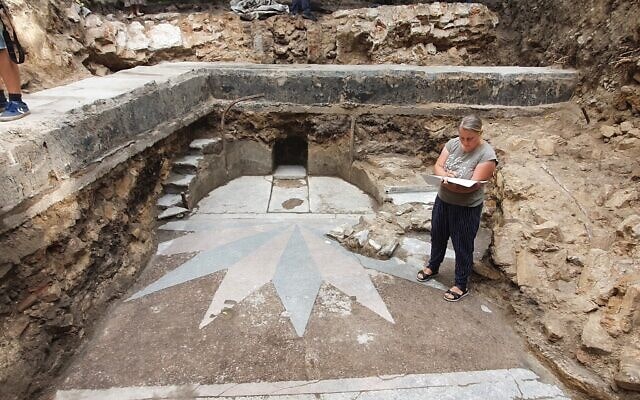The photograph captures a detailed scene of an archaeological excavation site. Central to the image is a woman, dressed in a light gray shirt and jeans, intently reading a piece of white paper. Her pale skin suggests she is Caucasian, and she appears to be deeply engrossed in her task. The site itself is a hollowed-out rock formation, predominantly brown and gray in color, with a complex, tunnel-like structure at its center. Surrounding the excavation site are distinctive spike-like structures, and the ground below features a unique design reminiscent of sun rays, tinted with light blue and gray hues. Partially visible in the top left corner of the image are the legs and blue sneakers of another individual, who seems to be standing on a higher level within the excavation area. A cement wall borders part of the site, emphasizing the methodical nature of the archaeological dig. Overall, the scene vividly conveys the meticulous and engrossing nature of an archaeological expedition.